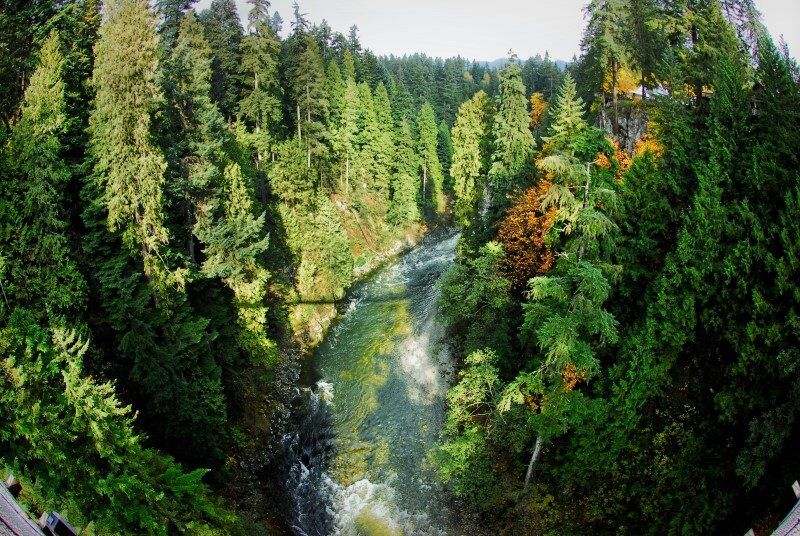The image portrays a serene wooded area, likely a state park, dominated by an abundance of tall, lush pine trees stretching to the horizon in every direction. In the center, a 20-foot-wide river winds its way downstream through the forest, its rushing waters creating rapids and white waves that reflect the surrounding greenery. The sunlit bank on the left middle side of the image reveals a brown soil surface adorned with green shrubs, while to the right, a rock bluff rises prominently. The scene is captured from a viewing area marked by a guard rail in the bottom corners, suggesting a designated spot for visitors to admire the natural beauty. Despite its photographic realism, the vivid details and textures imply the image might be a skillfully rendered painting.